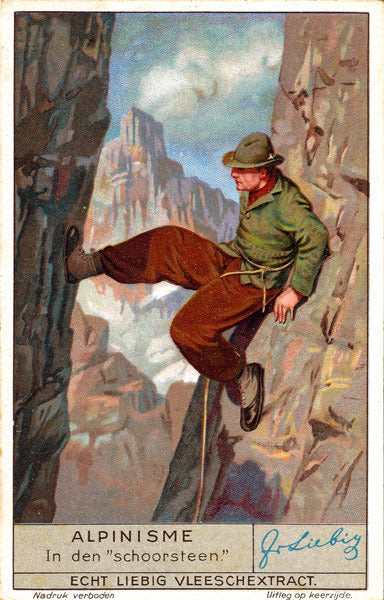The image depicted is an old postcard, likely from 50 to 100 years ago, showcasing an early rock climber or mountain explorer. The climber is prominently positioned in the center, using his right leg to steady himself by pressing against the left wall of a narrow ravine. He is wearing a green hat with a rim, a green jacket, baggy pants, and brown boots. A rope tied around his waist dangles between his legs. The scene, painted in a watercolor or similar style, features steep rock walls in the foreground, with taller mountains and a cloudy blue sky in the background. The predominant colors include brownish-red, green, yellow, beige, and blue. Below the climber is a caption, possibly reading "Alpinisme," suggesting a focus on mountaineering. This text is accompanied by additional writing in an unfamiliar foreign language, which might be Dutch, Swedish, or German, and a signature in blue ink at the bottom right corner.